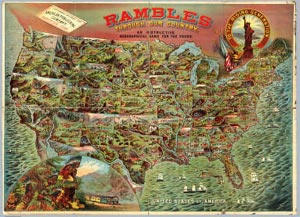The image depicts an aesthetically styled map of the contiguous United States, characterized by a visually artistic design rather than geographical accuracy. It is adorned with various images, including mountains, roads, and trains, set against a predominantly green backdrop to symbolize natural landscapes, possibly with plant and landmark motifs. The map is titled "Rambles Through Our Country," although much of the accompanying text is pixelated and difficult to discern. Notably, it excludes Alaska and Hawaii. At the bottom left, there is a circle featuring an image of Native Americans observing a passing train, and the top right corner contains another circle with the Statue of Liberty, encircled by the phrase "To Our Rising Nation." Additionally, what appears to be a license plate, possibly reading "Washington," is located in the top left corner. The map bears the aesthetic of a vintage poster, possibly from the 1940s, evoking a nostalgic portrayal of early American settlement days.